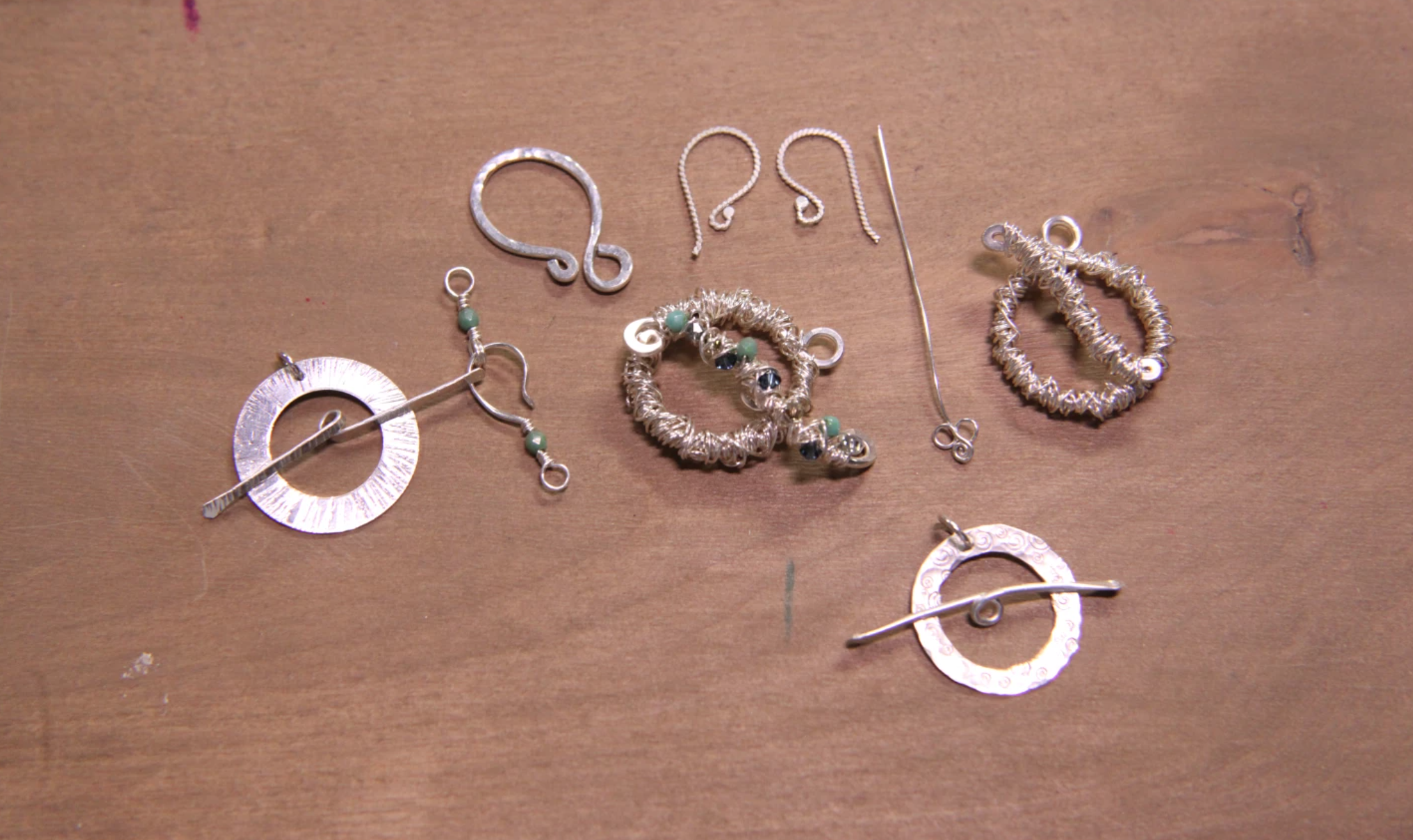The image showcases a variety of jewelry pieces arranged on a light brown wooden desk. Central to the arrangement are several unique metallic bracelets. One of these stands out with its intricate design of delicate metal wires, threaded with green and blue beads, and interspersed with swirling metal decorations, forming a circular shape reminiscent of a ring. Adjacent to it is a similar bracelet that excludes the beads, focusing solely on the polished metal swirls.

Among these, there are also distinct metal rings with swirls and circular cutouts, incorporating flat metallic rods. One notable piece appears to be a circular silver pendant, potentially an earring, adorned with turquoise beads at its ends, hanging from a fine wire. Another piece looks like a long, skinny metal rod in silver, adding to the eclectic collection.

The display also includes pieces that resemble horseshoes and gold-string-wrapped rings with a mixture of turquoise and dark blue beads. One particular pendant is marked by silver squiggly lines and features a narrow silver stick running through its center, extending beyond its circular boundary and anchored by a circular middle section. The entire assortment, reflecting a blend of classic and modern aesthetics, is meticulously spread out on the wooden surface, inviting closer inspection of each component's craftsmanship and detail.